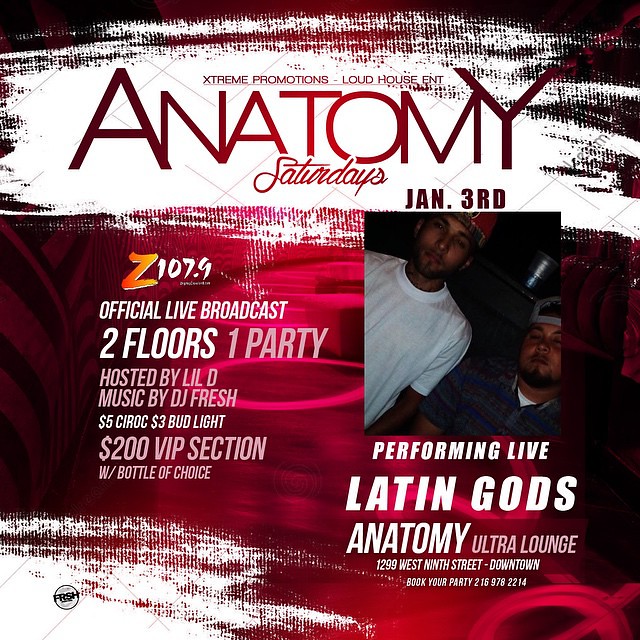The poster, predominantly red with white and black elements, advertises an event hosted by Extreme Promotions, Loud House ENT, and Anatomy. The title, "Anatomy Saturdays," is prominently displayed in a white strip with brushstroke effects at the top. The event is happening on Saturday, January 3rd at 1299 West 9th Street, Downtown. The text details that the Latin Gods will be performing live at L'Altre Lounge. Contact information for party bookings is provided: 216-978-2214. To the left of the poster, it announces a Z107.9 Official Live Broadcast, featuring two floors and one party hosted by Little D with music by DJ Fresh. It also mentions special offers including $5 Sirkak, $3 Bud Light, and a $200 VIP section with a bottle of choice. There is a small image on the left side showing two men in baseball caps, one in a white t-shirt and the other in a dark shirt, set against a red background.